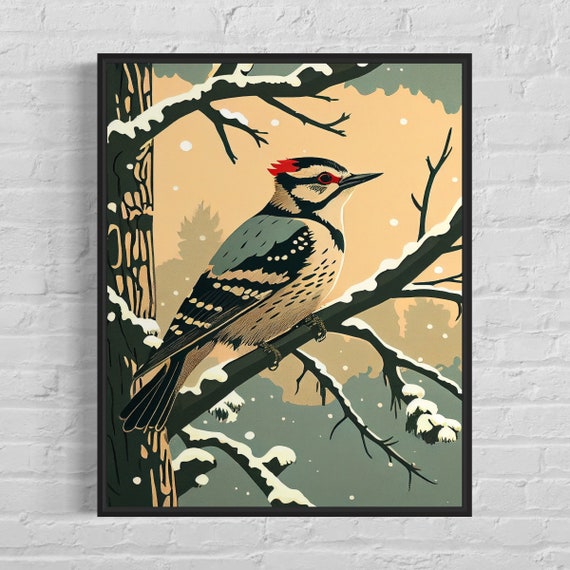The image features a meticulously framed illustration of a woodpecker perched on a snowy tree branch, all set against a beige and grayish background that creates a wintery atmosphere. The art, which has a cartoonish and computer-generated appearance, is framed in a slender black border and prominently displayed on a white, painted brick wall. The woodpecker itself is intricately detailed, with a white belly adorned with black spots and wings that are primarily a dark bluish-black with white stripes and dots. The bird's neck area features light blue feathers with black spots, and its head is marked by a distinct red crest and red spots near its sharp beak and eyes. The tree trunk on the left side of the image has a textured, bark-like appearance with beige patches, and multiple branches, all dusted with snowflakes, stretch out into the scene. The setting is further enhanced by snow falling gently around the bird, evoking a serene, wintry feel.